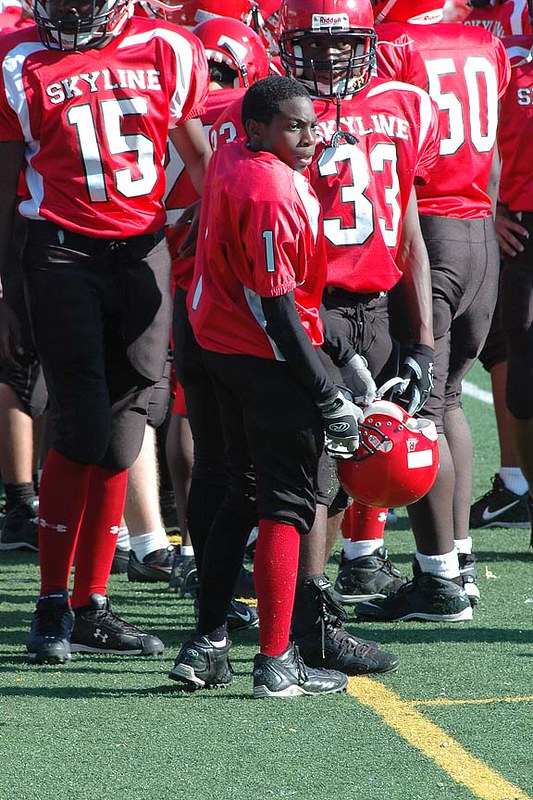The photo depicts a football team standing on an AstroTurf field, characterized by yellow and white lines. The players are all dressed in matching uniforms: red jerseys with white stripes that have "Skyline" inscribed on the front, along with black pants and black cleats. They are also equipped with red helmets and gloves. The image shows the players gathered closely, suggesting they might be on a break or during a timeout. Among them is a shorter African-American player who stands out; he has removed his helmet, revealing a younger face, and is looking off to the side at something outside the frame. He is wearing white gloves and a long-sleeved garment beneath his red jersey. The team appears to be at a pause, awaiting their return to action on the field.